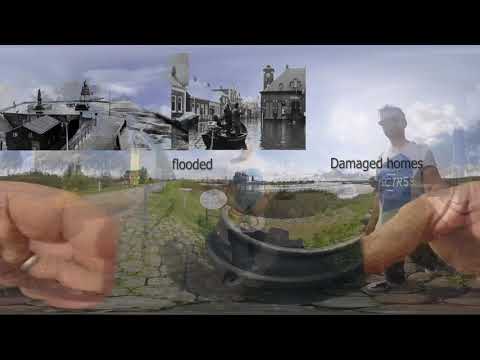This image features a collage-like, photoshopped scene with a transparent overlay effect. At the center, a Caucasian man wearing a white shirt with blue accents and sunglasses appears to be holding a camera. He is walking along what looks like a subtly distorted, cobblestone path or cracked asphalt road. Superimposed over this scene is text that reads "Flooded Damaged Homes," suggesting a flood disaster. In the top left and right corners, there are blended, black-and-white images that depict an old village with people navigating through floodwaters in boats. The overall composition has a messy and layered feel with scattered objects, including a hand with a ring on the far left. The colors predominately include shades of blue, white, black, gray, and tan, creating a somewhat ghostly atmosphere. The direction and intention seem to hint at a transition or overlay of past and present scenes of flood damage, possibly intended for a presentation.